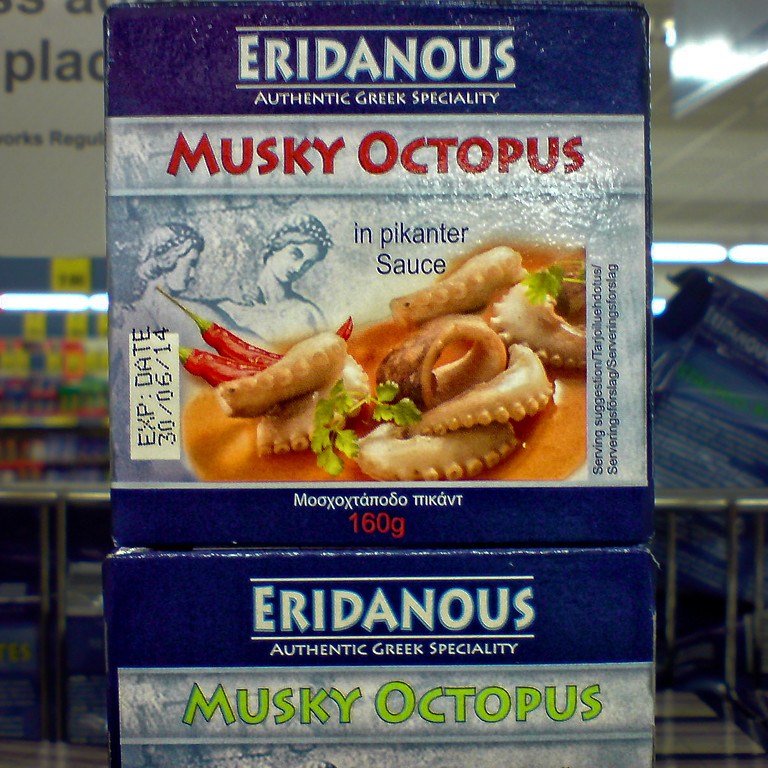The image displays an advertisement for a food product package labeled "musky octopus." At the top, in white text, it prominently features the brand name "E-R-I-D-A-N-O-U-S," followed by the description "Authentic Greek Specialty." The central area of the package highlights images of octopus in sauce, garnished with two sprigs of parsley and two chili peppers, suggesting a mildly spicy flavor. The phrase "musky octopus" is written twice: first in red, near the top of a marble-like design that evokes classical Greek aesthetics, and again in bright green at the bottom. Further details include blue text on a cream-colored bar indicating an expiration date of 30-06-14 and a weight of 160G. In the background, there is a hint of a store environment, with the package appearing to be placed in a wire basket or grocery cart. Additionally, there is some Greek text at the bottom of the image that is not legible.